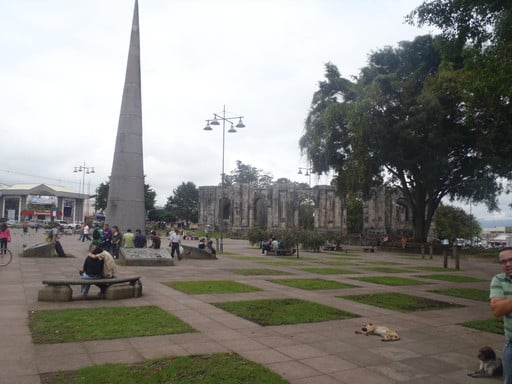The photo captures a bustling town square that doubles as a park, with a detailed and varied landscape blending historical and natural elements. The expansive plaza is laid out in a grid pattern with brown pavers interspersed with green grass squares. Towards the lower right corner, a man and his two dogs—one sitting, the other lying down—can be partially seen. On the left side, a cement bench hosts a couple, one person’s arm affectionately around the other, both facing away from the camera. Dominating the central area of the square is a prominent, cone-shaped monument or statue around which numerous people are gathered, suggesting its significance as a focal point or tourist attraction. In the background, to the right, ancient ruins resembling Greek architecture and what appears to be a visitor center offer a glimpse into the historical depth of the location. A large, venerable tree, which seems to have been standing for a long time, occupies the upper right portion of the image, providing a natural canopy over the scene. This picture vividly blends human activity with historical and natural elements, creating a rich tapestry of interaction and environment.